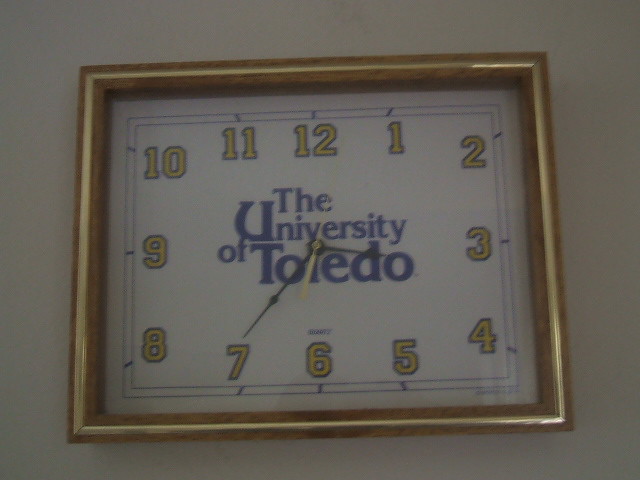This analog clock, square or slightly rectangular in shape, proudly represents the University of Toledo. School spirit shines through in the design, featuring numbers adorned in gold with blue trim, the university's official colors. The time reads approximately 3:35. The clock's sophisticated wooden frame adds an element of elegance, further enhanced by a gold-inlaid metal centerpiece, albeit more likely a gold-colored material, emblazoned with "University of Toledo." This eye-catching timepiece is mounted on a pristine white wall, appearing perfectly suited for a place of prominence, such as the university's admissions office.